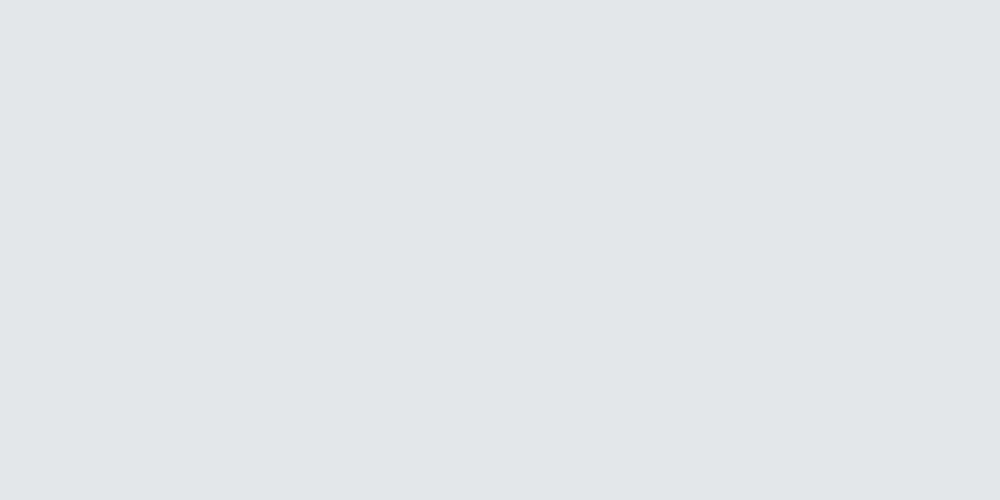This is a rectangular image of a light gray box, predominantly brighter on the right side and featuring darker shadings near the upper left-hand corner, transitioning down to the lower left-hand corner. The horizontal length of the box is significantly greater than its vertical height, and there are no discernible text or markings to provide context or explanation. The image appears plain, with no background elements or faded details that might suggest an underlying meaning or purpose. It is unclear if this presentation is intentional or if it might be an oversight or error.